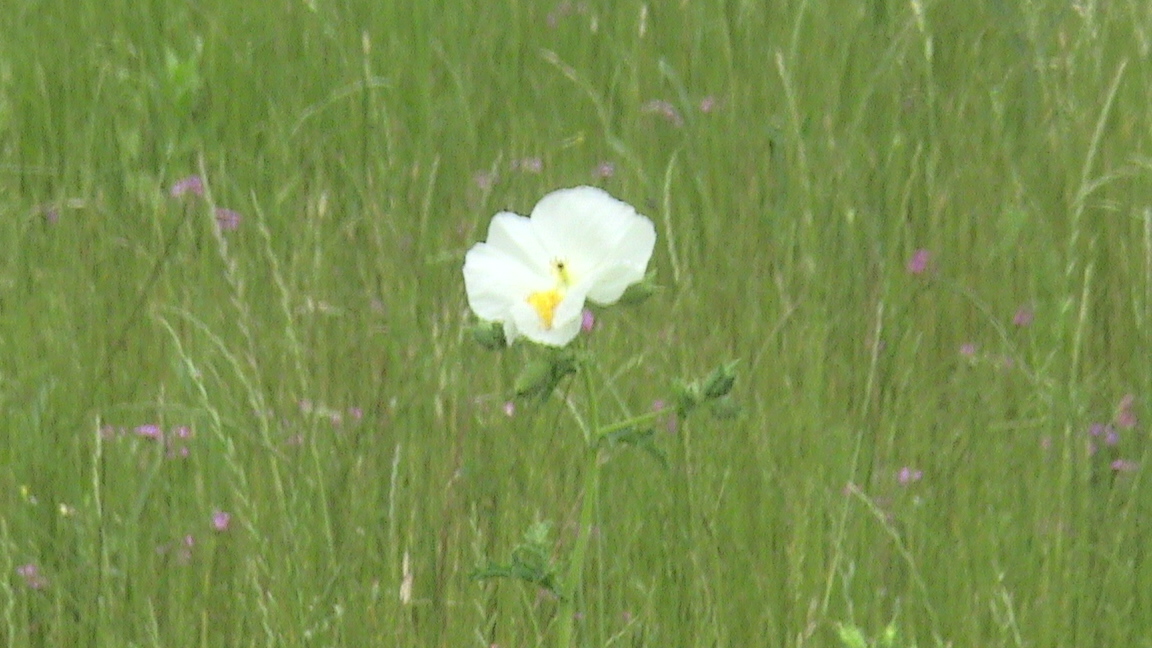This horizontally aligned, blurry photograph features a vivid outdoor field with a central focus on a single prominent white wildflower. The flower, reminiscent of a fluffy carnation with cloud-like petals, has a yellow center and a small brown seed at its core. It is attached to a thin, long green stem, which branches out with several smaller buds yet to bloom. Surrounding this central flower are numerous tall blades of green prairie grass, interspersed with small purple wildflowers that might be violets. The greenery extends upward, fading into a blurry background where fewer purple flowers are visible.